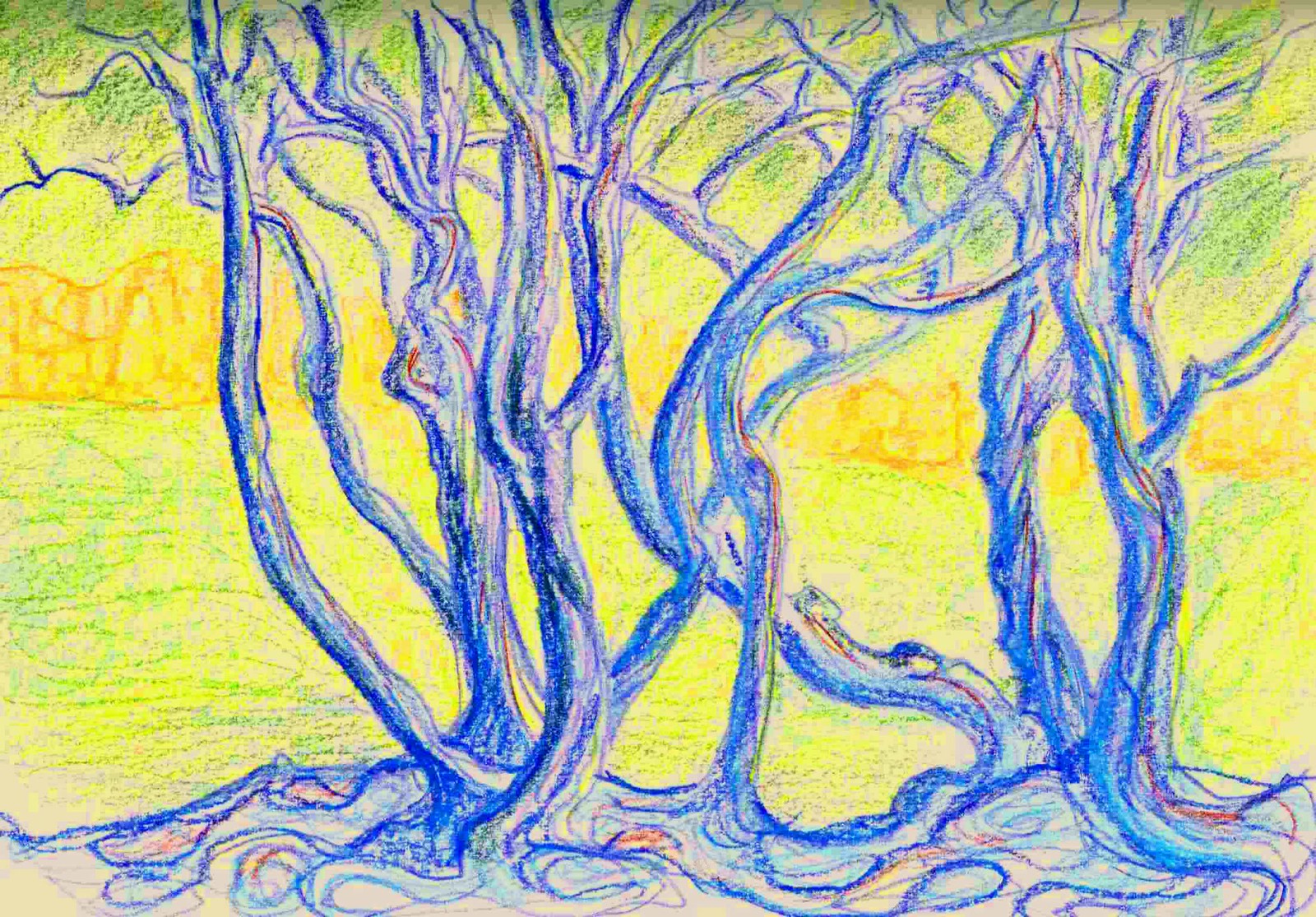This abstract-style drawing boasts a vibrant and colorful palette featuring greens, yellows, purples, and blues. The background is a vivid bright green, interrupted by a striking yellow-orange stripe that transitions back to a bright yellow-green hue towards the top. The image showcases tree-like forms with swirling, wave-like trunks and intertwining branches that evoke the appearance of vines. These trunks are rendered in purplish-blue tones accentuated by red lining, creating an illusion of them melting into red roots embedded in the ground below. The entire composition exudes a dynamic energy and captivating vibrancy.